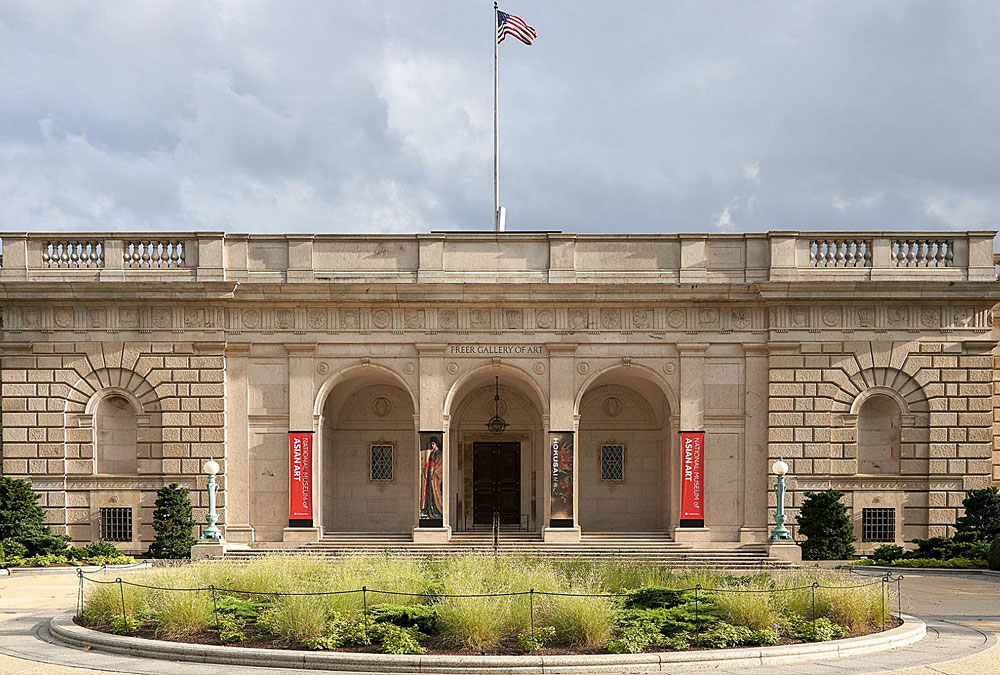The image captures the front of the Freer Gallery of Art, prominently featuring the gallery's name engraved on the facade. This one-story building has a classic brick architecture with a light tan stone appearance and is adorned with a balcony at the top, characterized by stone railings. In the very center of the building, a tall silver flagpole with an American flag fluttering in the light breeze stands out against the overcast, light gray-blue sky.

The entrance, which is right at the middle of the building, is framed by three elegant archways with curved tops. The central archway serves as the main doorway, featuring dark double doors and a series of low stairs leading up to it. Banners drape down from each archway, with the central banner reading "Asian art" in red letters.

In front of the gallery, there's a circular driveway lined with a small garden area. This garden is enclosed by a concrete frame and filled with green bushes, shrubbery, and strawberry plants. The overall scene conveys a serene and dignified atmosphere, typical of a prominent art museum.